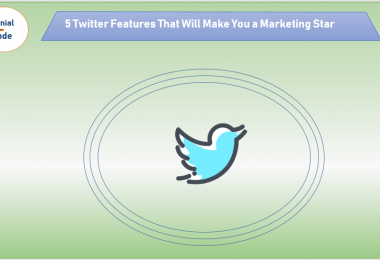The image is a screenshot of a website designed to offer marketing advice specifically for boosting your business using Twitter. It is rectangular and landscape-oriented, slightly longer than it is tall, with a green background that fades to white in the center before transitioning back to green. 

In the upper right-hand corner, there is a partially visible white speech bubble outlined in orange, containing blue text separated by an orange line; the readable portion of the text includes "N-I-A-L" followed by an orange line and "D-E." At the top of the image, a blue trapezoid-shaped ribbon displays the text "5 Twitter features that will make you a marketing star" in white font.

Centrally located is an oval composed of three concentric blue lines, inside which is a black outline of the Twitter bird icon. The bird is primarily filled with blue paint but is noticeably off-center, revealing some of the white background, which may be an intentional design choice or an error.

Overall, the webpage appears to be focused on providing tips and strategies to enhance your marketing efforts on Twitter.